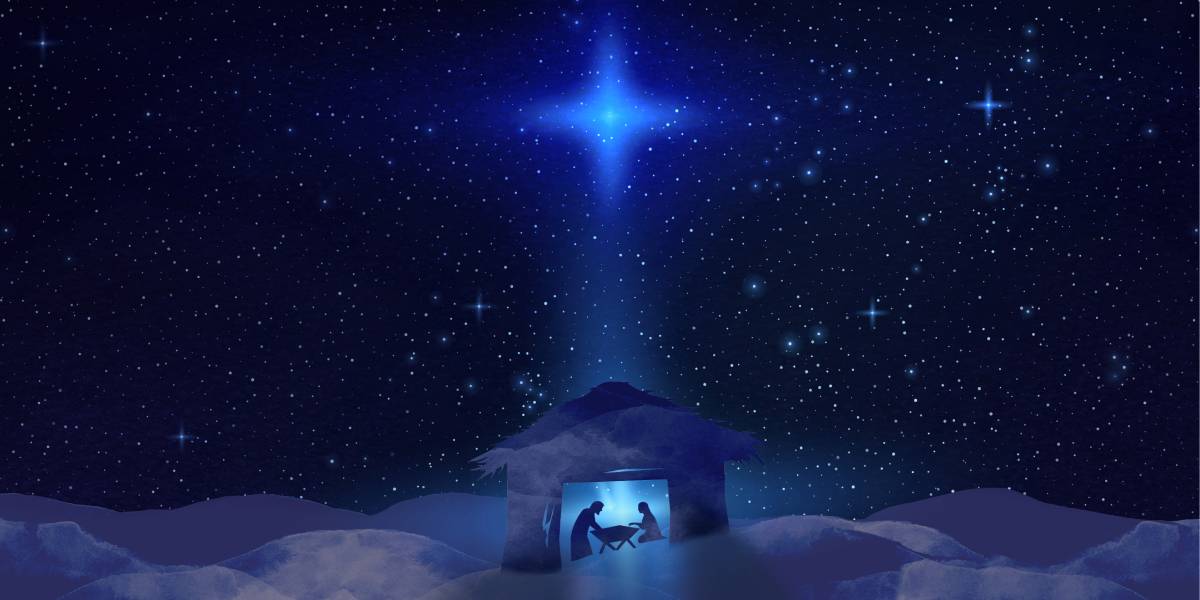The image beautifully captures the nativity scene, set against a mesmerizing night sky in hues of deep blue, midnight blue, and purple. The sky is dotted with numerous twinkling stars, but one exceptionally bright star stands out prominently in the center, casting a radiant beam of light downwards. This luminous star is directly above a modest thatched hut nestled among sand dunes. Within the hut, the silhouettes of a kneeling woman and a standing man can be seen, both reverently gazing into a crib placed between them. The light from the star illuminates the crib, emphasizing its significance in the serene and mystical setting. The overall palette includes shades of blue and black, with subtle clouds adding to the ethereal atmosphere.